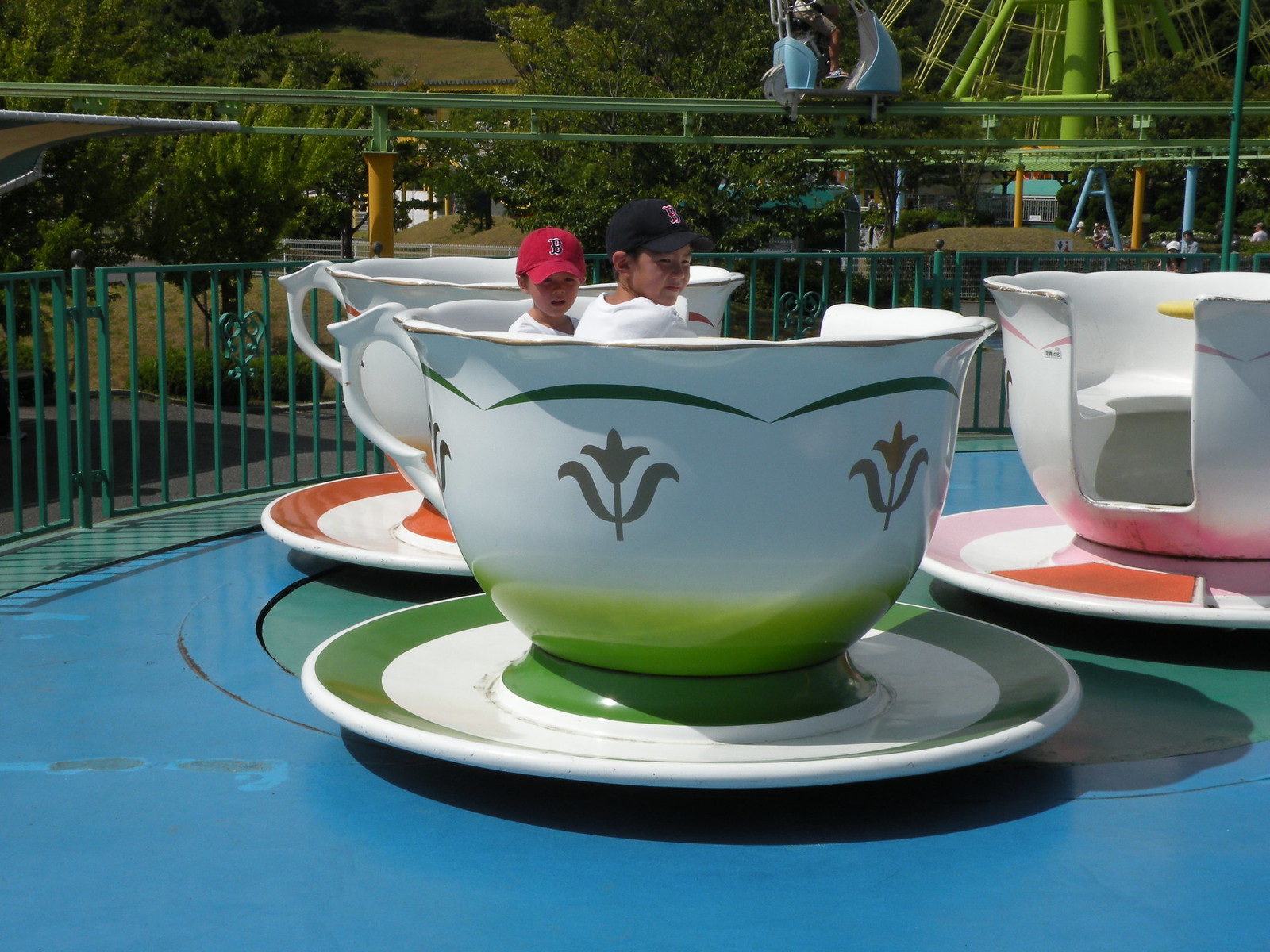This vibrant photograph captures a lively teacup ride at an outdoor amusement park, possibly Walt Disney Amusement Park, set against a backdrop of lush green hills and verdant trees. In the foreground, a large white teacup with green flower designs and a green rim sits on a matching white plate with green stripes, all perched on a bright blue floor. Inside this teacup are two Caucasian boys, each clad in a white t-shirt; one wears a navy blue cap adorned with an insignia, and the other sports a red cap with a similar marking. The boys appear to be looking directly at the camera. Surrounding the scene are additional teacups in the background, suggesting the ride's circular arrangement. Off to the right, a yellow metal structure, likely a ferris wheel, is partially visible, adding to the festive atmosphere. Moreover, a grayish-brown track with a yellow support pillar runs from left to right in the mid-background, with a whitish vehicle visible on it, contributing to the bustling carnival ambiance.